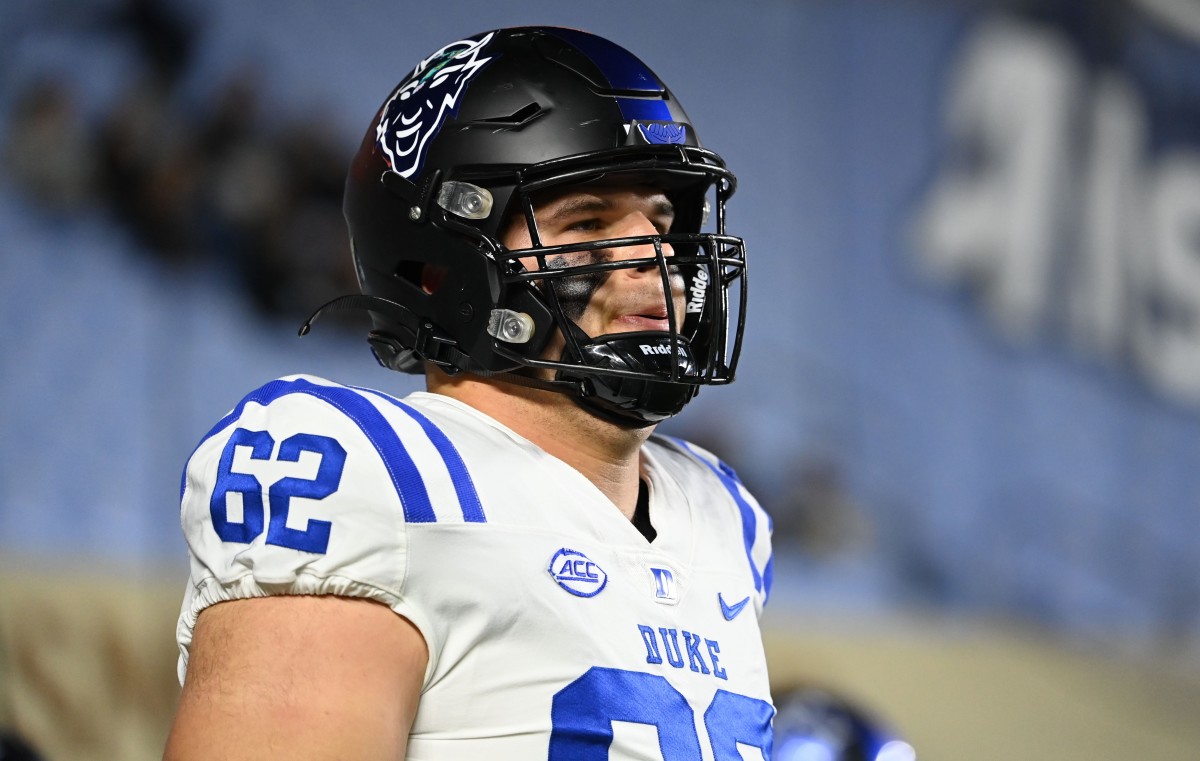The image shows a close-up, three-quarter view of a Caucasian Duke football player who is gearing up at what appears to be an unspecified stadium, characterized by a heavily blurred background with shades of blue, tan, black, and white. He wears a black helmet adorned with a devilish face on the side, obscuring much of his face, although black streaks for glare reduction are visible beneath his eyes. His expression is serious, with pursed lips as if blowing out or breathing heavily. The player is clad in a white jersey marked by blue details, including two stripes on each shoulder, a large 'D' at the neckline, and the inscription 'Duke' prominently across the chest. His jersey also features the number 62 on the sleeves and a small circle with letters on the right chest, while a checkmark symbol appears on the left. The lighting captures the clarity of his figure against the indistinct background, accentuating the intensity and focus of the moment.